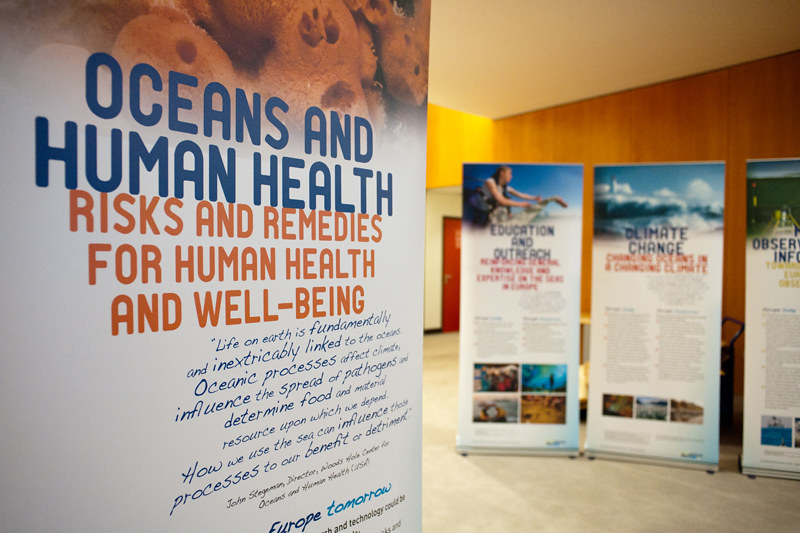This image depicts an indoor setting, likely a museum or an event space, with several vertical posters arranged on stands. The flooring consists of cream-colored tiles, and the room is well-lit with a creamy ceiling and brown and yellow walls. In the background, a red door is partially visible, enhancing the warm ambiance.

On the left side of the image, a prominently displayed poster titled "Oceans and Human Health" is detailed with a photograph of stones or objects at the top. The poster includes the subheading "Risks and Remedies for Human Health and Well-being" in orange. The primary text in various blue fonts explains the critical link between life on Earth and the oceans, noting how oceanic processes affect climate, determine resources, and spread pathogens. It also mentions that human use of the sea can significantly impact these processes, either beneficially or detrimentally. This poster credits John Stemmen, Director of the Woods Hole Center for Oceans and Human Health, USA, and bears a logo with the words "Europe" and "technology."

To the right, additional posters discuss topics such as "Education and Outreach" and "Climate Change," although their details are blurry and hard to decipher. The posters contribute to a thematic arrangement around climate-related issues and human interaction with the environment. The overall color palette of the image includes shades of white, blue, orange, light blue, black, brown, and tan, creating a cohesive yet vibrant visual narrative.